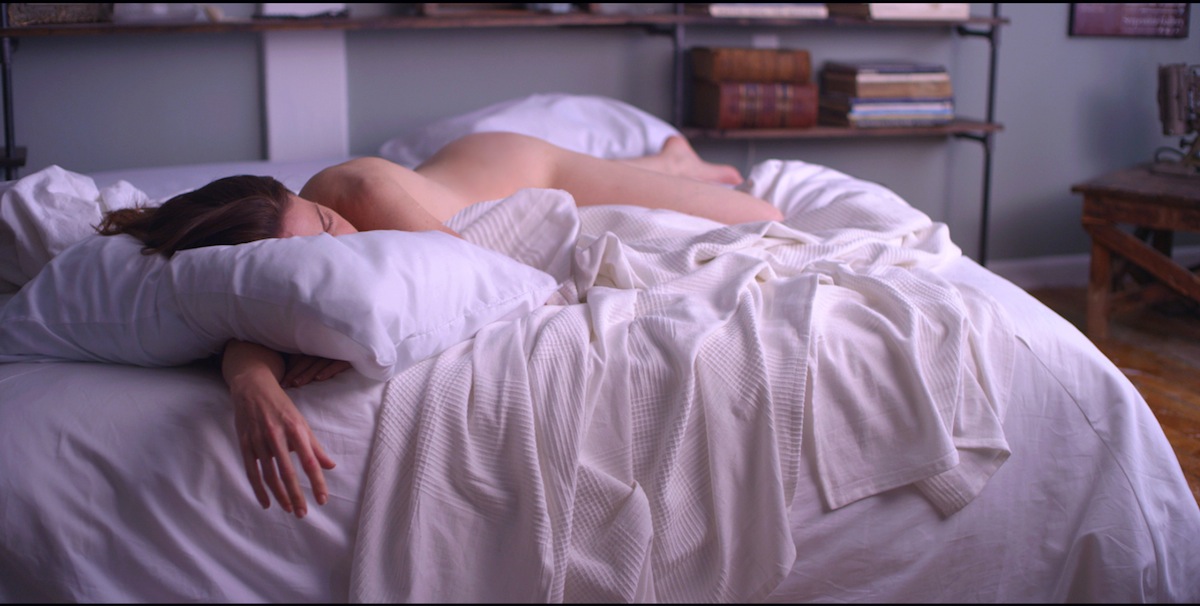In this detailed bedroom scene, a nude woman with brown hair lies asleep on a bed positioned to the left. She is lying face down with her chest on the bed, her head resting on a white-cased pillow. One of her hands is tucked under the pillow, while the other hand drapes off the side of the bed. Positioned at her feet is another pillow. The bed itself is dressed in white bedding, including both the bedsheet and a nearby blanket. The room features a blue wall adorned with white-framed pictures and a wooden shelf holding an assortment of books. On the right side of the image stands a wooden table, which supports an unidentifiable device. The floor is composed of brown floorboards, adding a warm tone to the scene.